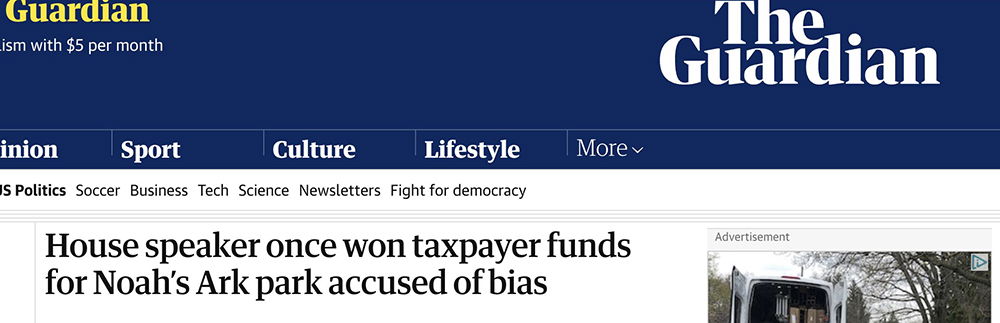Screenshot from The Guardian website: 

At the top left corner, there is a gold bar containing "Guardian" and "$5 per month for journalism." On the top right corner, the logo "The Guardian" is displayed in large letters. The left side of the page is slightly cut off, but several navigation topics are visible across the top, including "opinion," "sports," "culture," "lifestyle," and a drop-down menu labeled "more."

Subtopics listed include "US politics," "soccer," "business," "tech," "science," and "newsletters," with an additional mention of "fight for democracy." A couple of gray lines create a border, leading to the headline of an article titled, "House Speaker once won taxpayer funds for Noah's Ark Park accused of bias."

To the right side, there is a small box labeled "advertisement," directly above an image that appears to show the back of a delivery truck, potentially an Amazon truck, accompanied by surrounding trees.